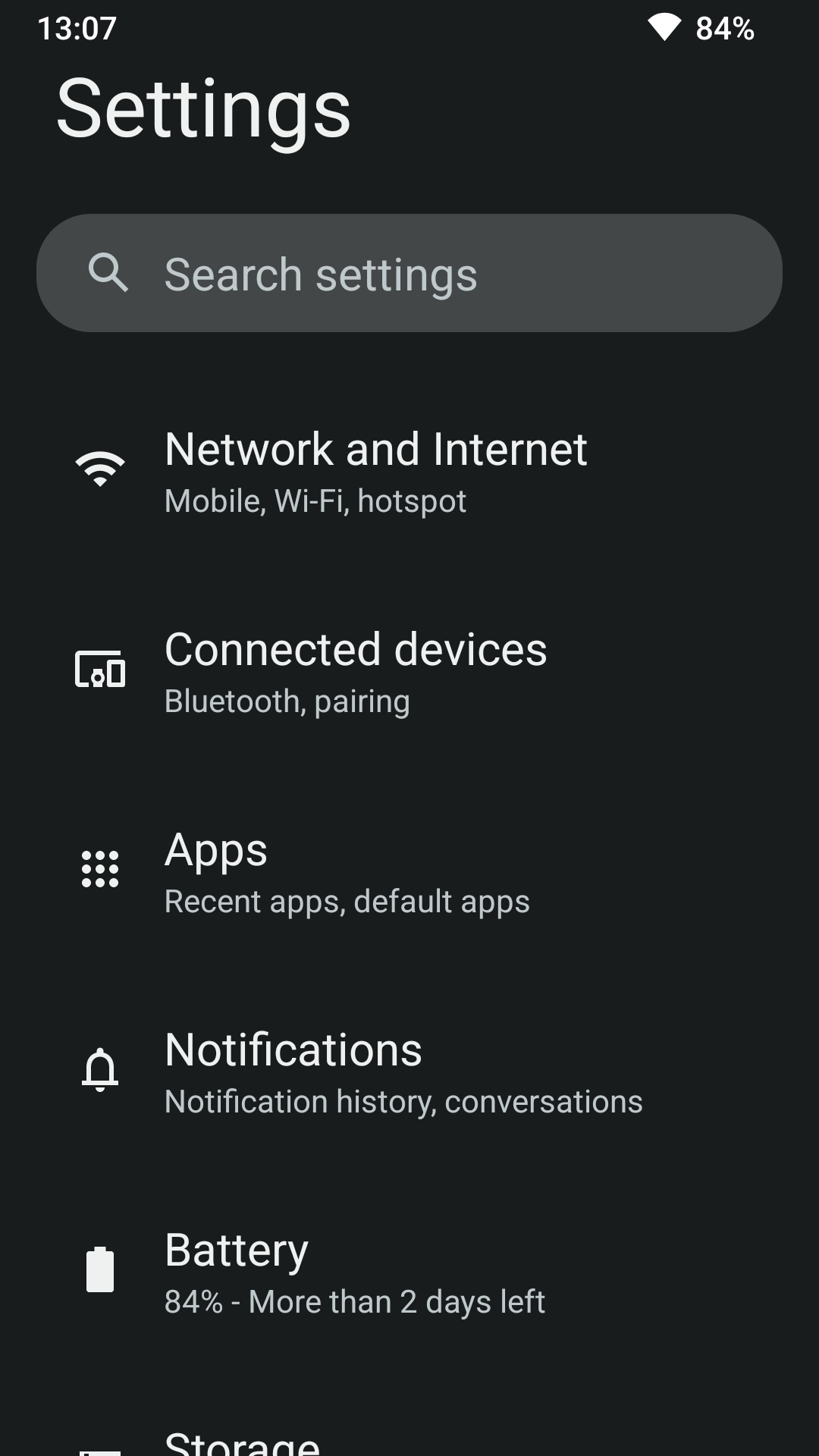The image displays a smartphone screen showcasing the "Settings" menu in dark mode. The background is black and the text is written in white for enhanced readability. 

At the top left corner, the text "Settings" is prominently displayed. Directly below this, there is a search bar with the placeholder text "Search Settings" and a magnifying glass icon on the left, indicating its function.

Following the search bar are various settings categories, each accompanied by a descriptive icon on the left. The categories are listed in the following order:

1. **Network and Internet** - The description includes "Mobile, Wi-Fi, Hotspot," with a Wi-Fi icon symbolizing different network options.
2. **Connected Devices** - Described with "Bluetooth, Pairing," and depicted by an icon featuring a tablet, watch, and smartphone.
3. **Apps** - This section mentions "Recent Apps, Default Apps," and is represented by an icon with nine small white dots.
4. **Notifications** - Includes "Notification History, Conversation," and is illustrated by a bell icon.
5. **Battery** - Indicates that the battery is at "84%, more than two days left," with a full battery icon showing the charge status.
6. **Storage** - Located at the bottom, this category is marked by a storage disk icon, detailing storage information.

All icons are drawn consistently in height and are positioned to the left of their respective text descriptions. This detailed layout provides a comprehensive overview of the main settings accessible on the smartphone.